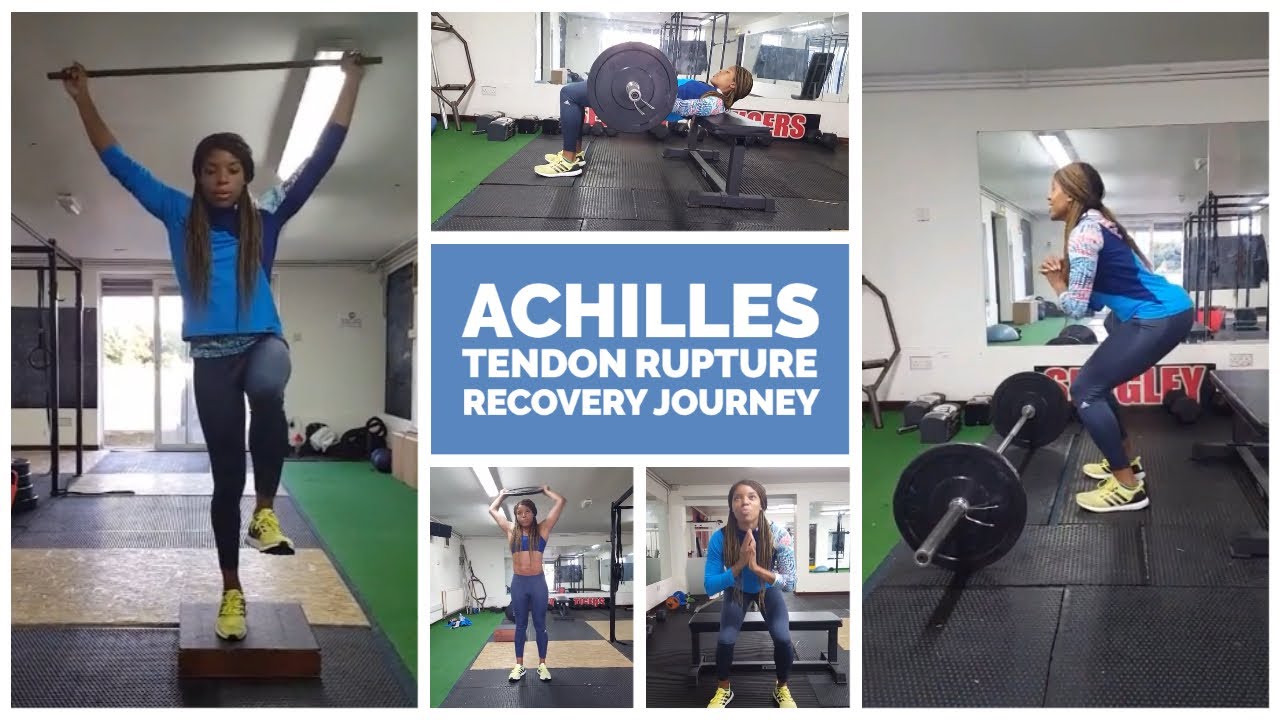The image showcases a black woman with long brown hair at a gym, working out in various exercises as part of her Achilles tendon rupture recovery journey. She is depicted in five separate photos, each capturing a different workout. In the images, she wears a blue long-sleeve shirt and blue leggings, though her outfits vary slightly. She consistently wears bright yellow neon sneakers. The exercises include lifting weights, holding a cane horizontally while stepping forward or using a stepping block, doing squats, and pressing a larger weight above her head. Each photo highlights her determination and progress in recovery.